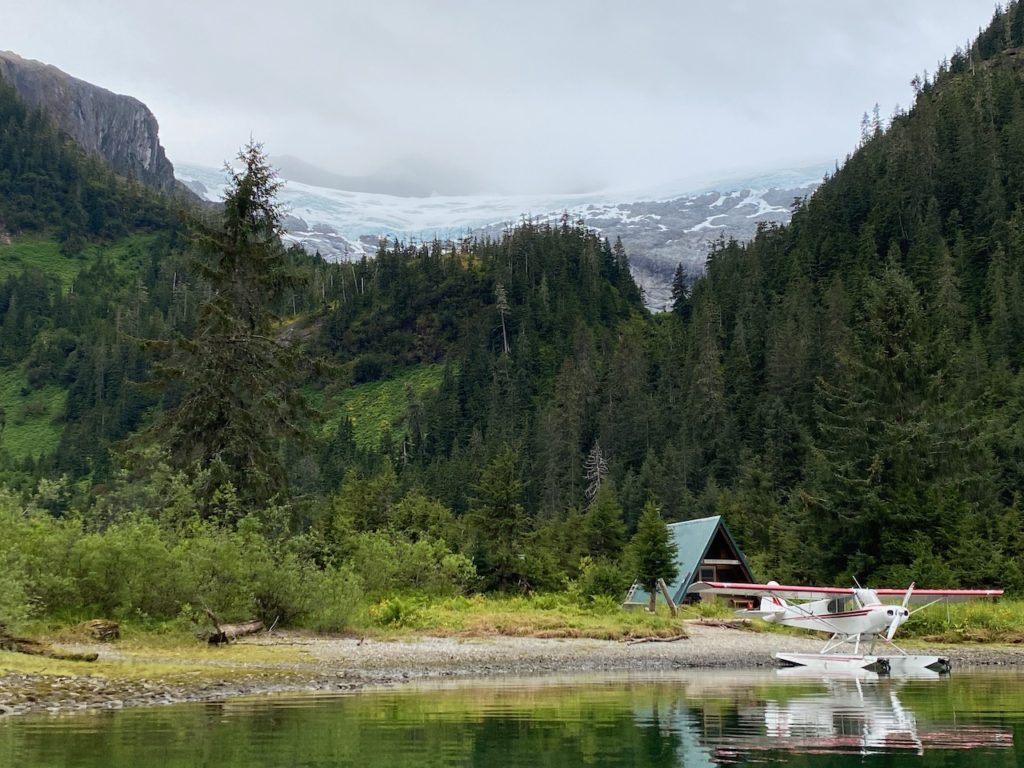A horizontal, rectangular photograph showcases a calm lake bordered by forested hills and towering mountains in the background. Dominating the lake's serene, green-reflected surface is a seaplane equipped with skis, gently floating. Just behind the plane stands an A-frame cabin with a green roof extending to the ground, its front characterized by a brown facade and a distinctive triangular shape. This picturesque scene is rich with diverse vegetation—pine trees and dense forests envelop the area, creating a lush, natural setting. The cabin and seaplane are nestled amidst this verdant landscape, flanked by rolling forest hills that lead to a dramatic backdrop of snow-capped, rocky mountains rising majestically against a gray sky, seamlessly blending into the scenery.